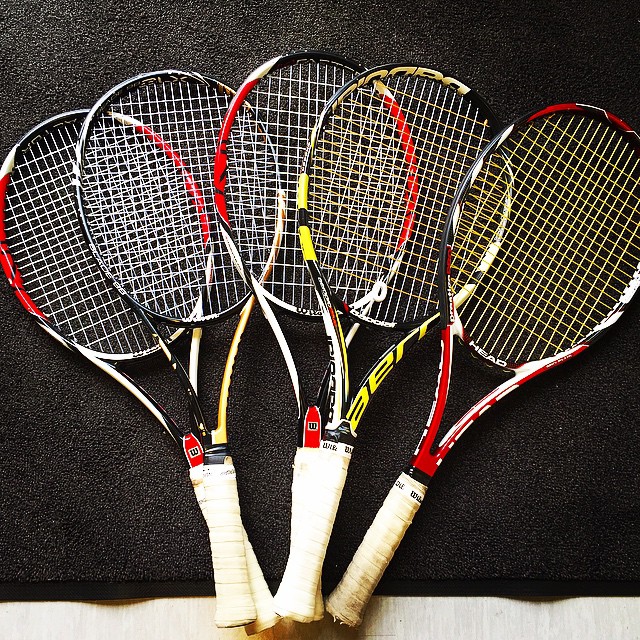This photograph showcases five tennis rackets arranged in an overlapping fan pattern on what appears to be a black foam mat, occupying most of the frame. The base of the rackets is clustered together at the bottom of the image, revealing their off-white gripped handles, some of which are visibly distressed or dirty. Each racket features a unique design: one red with yellow strings, one black and yellow with yellow strings, one red and white with white strings, one entirely black with white strings, and another black, red, and white with white strings. The frame of the image also includes a small portion of a light-colored wooden floor visible at the bottom edge. The background predominantly consists of a textured black surface, adding contrast to the image.